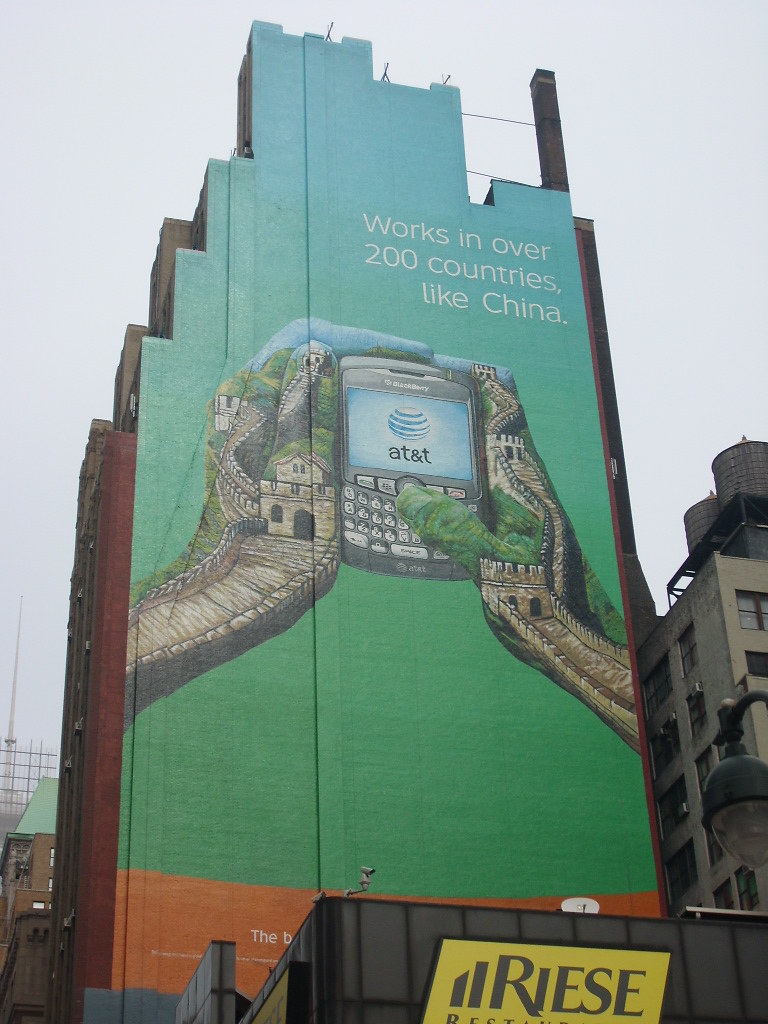Captured in this photograph is a striking advertisement displayed on the side of a multi-story building complex. Though the primary building is primarily constructed from tan-colored materials, a gray water tower crowns the structure, adding an industrial element to the scene. Adjacently, a black-colored building features a prominent yellow sign with black text spelling "R-I-E-S-E."

Dominating the right side of the composition is a tall, brownish-red brick building. Its architectural design incorporates a distinctive staggered effect near the top. The structure narrows progressively in a series of stepped recesses, creating a visually interesting tower-like appearance.

The focal point of the photograph is the advertisement itself, which spans the side of the brick building. The background of the advertisement is green, contrasting sharply with the white text that declares, "It works in over 200 countries like China." Central to the ad are two hands holding a classic gray-colored Blackberry device with a visible keyboard. An AT&T logo is subtly included on the device's screen. The imagery extends down the arms and across the hands, seamlessly incorporating an evocative depiction of the Great Wall of China, merging human and historical elements into a cohesive visual narrative.